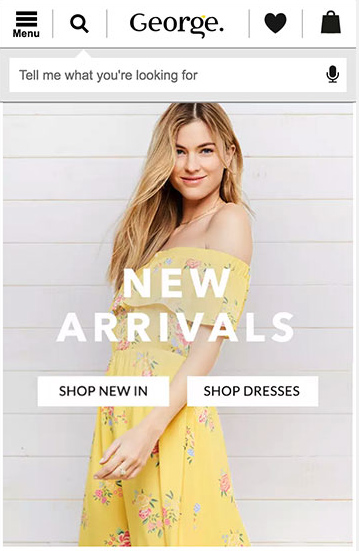The image appears to be a screenshot from a mobile phone displaying a shopping app interface. At the top of the screen, there is a navigation bar featuring several icons and text elements. On the left, there's a bolded menu icon represented by three horizontal lines with small spaces in between. To the right of this icon, a vertical separator line appears, followed by a magnifying glass icon indicating a search function. Another vertical separator follows the magnifying glass.

Next, the text "George" is displayed in a distinct font, with each letter clearly separated by spaces. The characters read "G-E-O-R-G," with a small yellow dot above the letter "G" and a period after the last letter. Following the text "George," there’s another vertical separator, a heart icon, another separator line, and an icon resembling a shopping cart or bag.

Beneath this navigation bar is a long rectangular search box with the placeholder text, "Tell me what you're looking for." This box has a slight upward-pointing element near the magnifying glass icon on its left side. On the right edge of the search box is a microphone icon, indicating a voice search functionality.

The central portion of the image features a smiling Caucasian woman with long hair, appearing to be in her late 20s. She is wearing a yellow spring dress adorned with floral patterns. Above her image, there’s a label stating, "New Arrivals." Overlapping the bottom of the image are two buttons: one that reads "Shop New In" and another that reads "Shop Dresses."